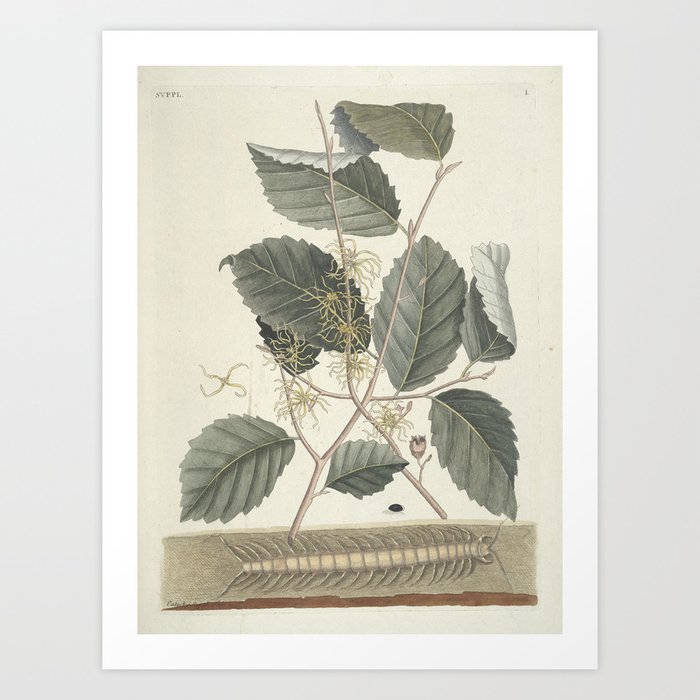This detailed botanical art print is set on a light blue background with a white matte frame. The muted, neutral tones of the print create a delicate and antique appearance. In the middle, dark greenish-gray leaves with pronounced veins are arranged to form a tower-like structure with intersecting branches. These branches feature thin limbs, some of which are adorned with small buds and the remains of dried flowers. The varying stages of the leaves' life add depth, with some leaves slightly turned or bent. Below the intricate foliage, a beige centipede-like figure, resembling a fossil, lies against the grey backdrop. The top left corner of the image includes some unreadable text, and there is a number one in the top right corner, contributing to the print's detailed composition.